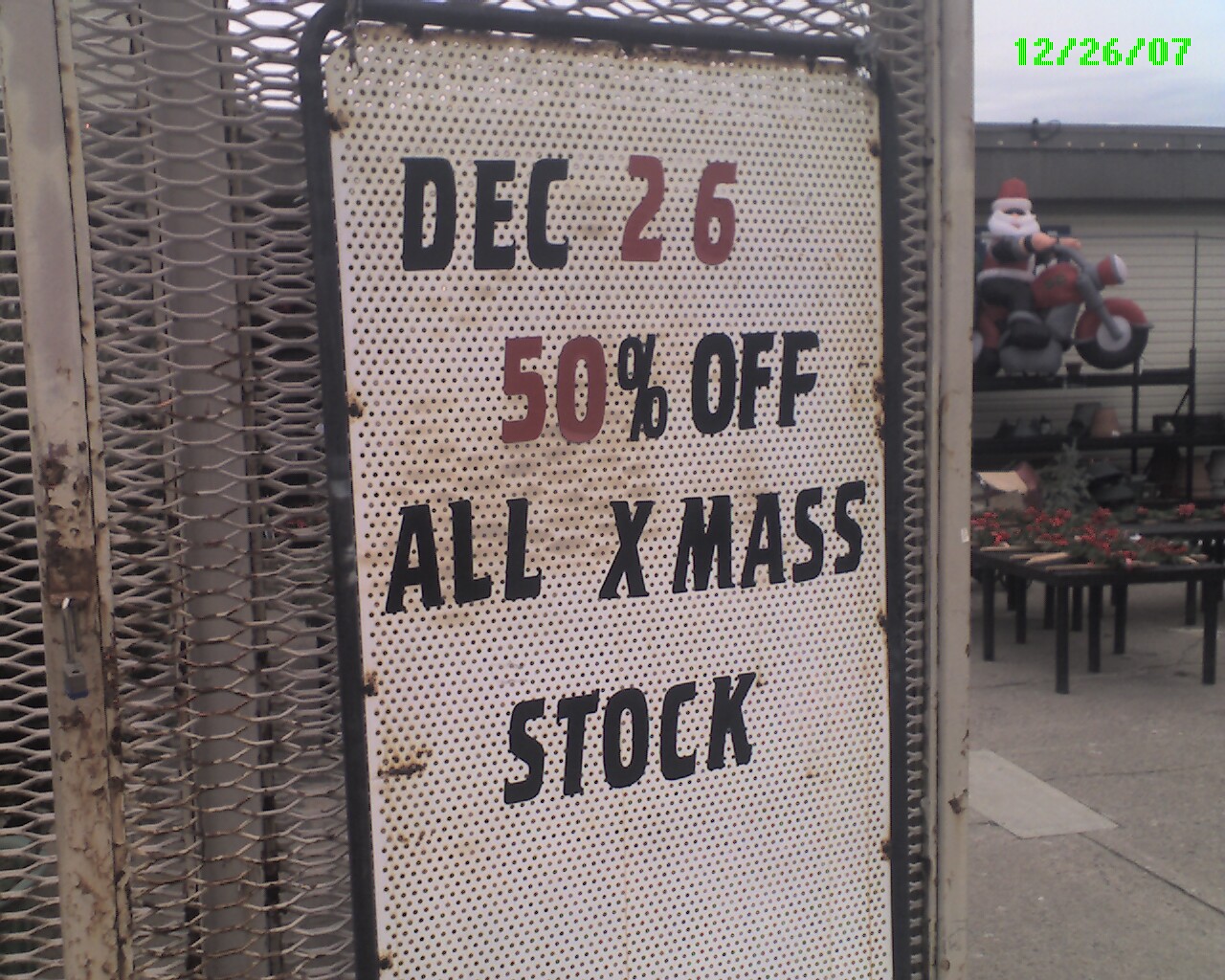The photograph captures an outdoor scene in front of a store, featuring a prominently displayed sign. The sign, mounted on a gray fence, has a white background peppered with tiny black perforations. It is rectangular with rounded corners, and its message is succinct: "December 26, 50% off all X-mas stock." The letters are in bold black, while the numbers are highlighted in vibrant red, drawing attention to the discount date and offer. Adding a festive touch, a large inflatable Santa Claus riding a motorcycle is visible in the background. The top right corner of the image also includes a neon green date stamp, reading "12-26-07."